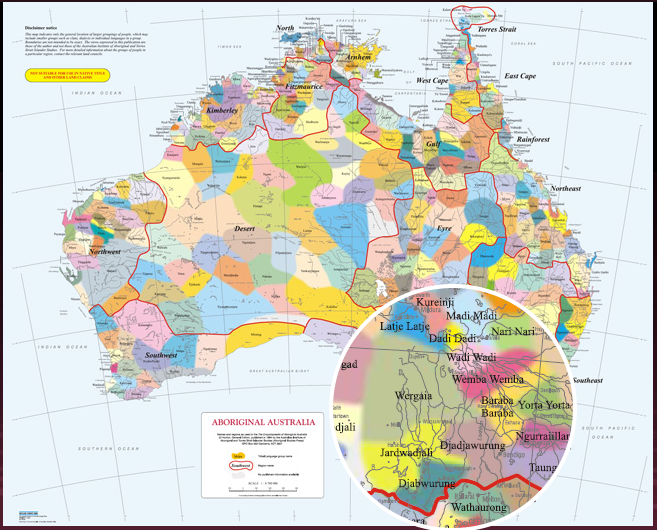This image depicts a detailed and color-coded map of Aboriginal Australia, focusing on the various groups of Aboriginal Australians and the cities they inhabit. The map features an array of colors including green, yellow, red, blue, pink, purple, light blue, dark blue, brown, white, navy blue, and darker red, each representing different areas for different groups. Notable cities such as Yorta and Wathaurong are highlighted within the detailed view. The title "Aboriginal Australia" is prominently displayed in pink letters within a white box at the lower part of the map. The surrounding ocean is shown in light blue, and a black box frames the entire image. Additionally, red outlines cluster around specific groups, further distinguishing the different regions represented on the map.